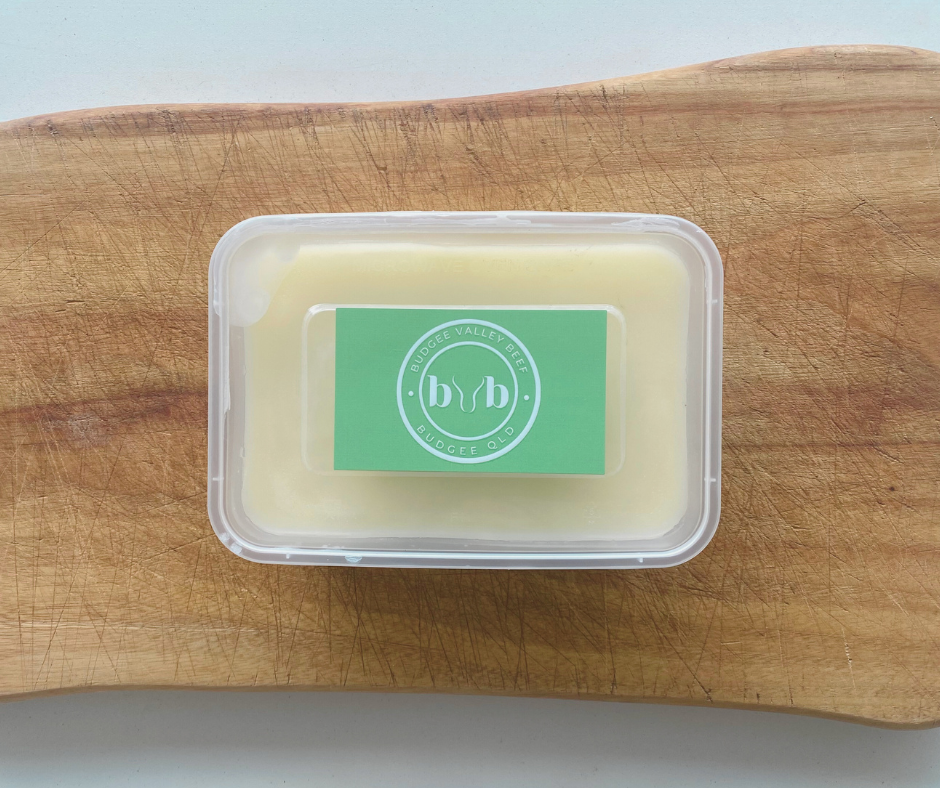The image depicts a light gray background, likely a countertop or table, with a prominent light brown wooden cutting board spanning its width. The cutting board bears numerous cut marks, adding texture to its surface. Placed centrally on the cutting board is a rectangular, clear plastic container filled with a solid, cream-colored or white substance, possibly beef tallow or fat. Affixed to the container is a light green rectangular label featuring a white circle within another white circle. The outer circle has the text "Budgie Valley Beef" at the top and "Budgie O Q L D" at the bottom. The inner circle contains a design resembling the letters "B V B," with the "V" mimicking cattle horns.